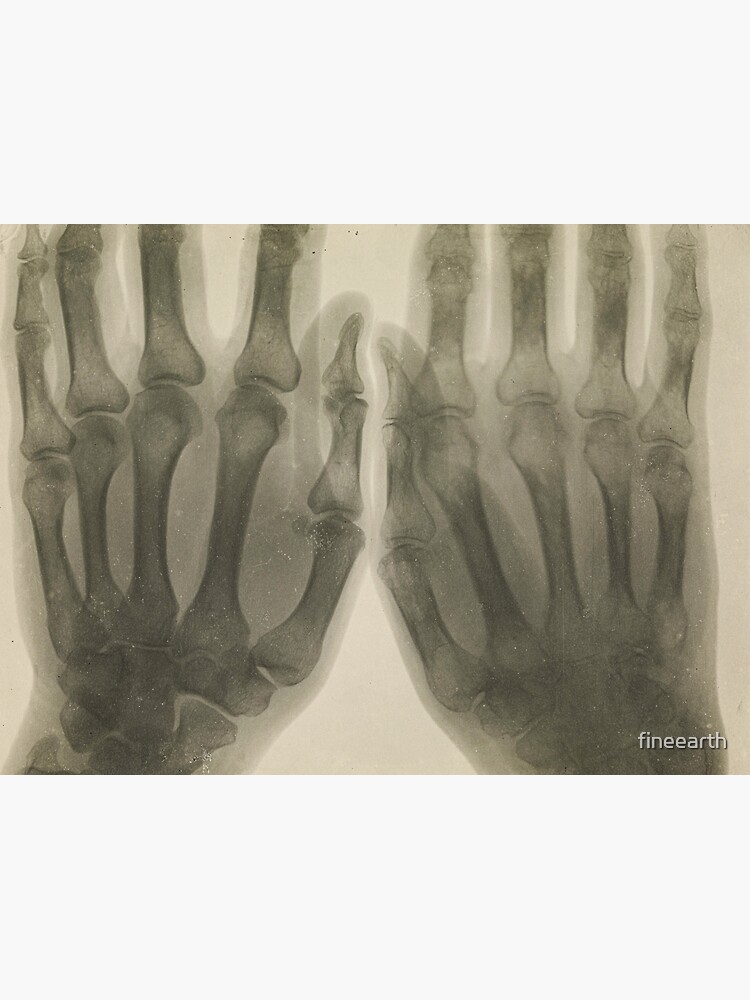This photograph features a monochromatic x-ray of two human hands side-by-side, palms down, positioned horizontally against a gray vertical background. The x-ray itself has a sepia tone with the darker areas appearing slightly gray-green and the lighter areas showing up as beige and light gray. Each hand is meticulously detailed, displaying the skeletal bones clearly, while the faint, ghostly outlines of flesh provide a translucent overlay. The hands' bones are distinctly darker than their connecting joints, and no fractures are apparent. The image cuts off just before the tips of the fingers, leaving the bones of the fingers, thumbs, and the cobbly collection of bones at the base of each hand visible. In the bottom right corner, white text with a slight gray outline reads "vintage wall art," enhancing the image's aesthetic appeal.